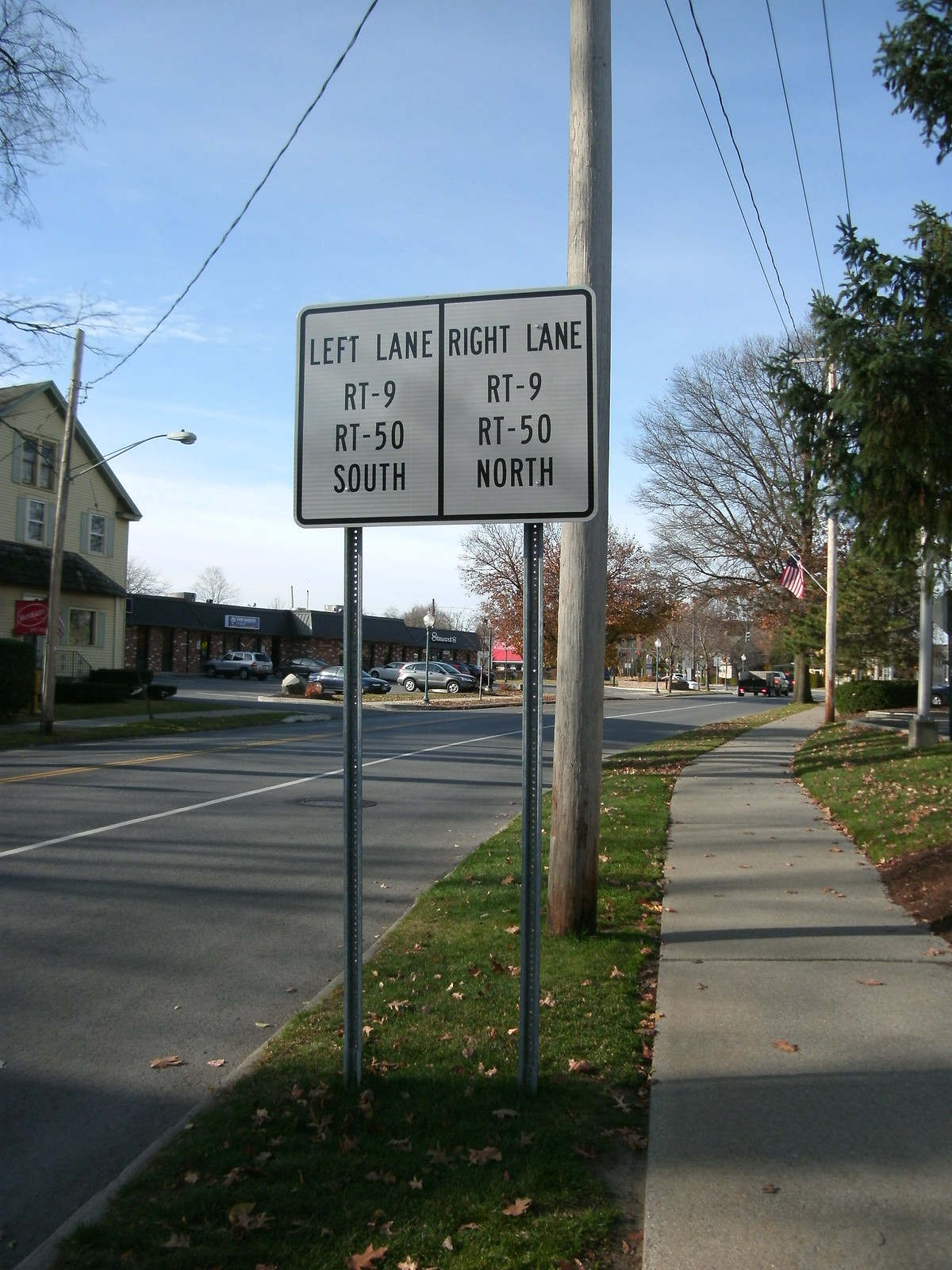The image captures a clear, well-maintained road with prominent signage directing traffic. Two road signs are mounted side by side, instructing drivers: the left lane for RT-9 and RT-50 south, and the right lane for RT-9 and RT-50 north. The signs are primarily white with black trim and are secured on a typical metal stake set in the grassy roadside. The pavement itself is unblemished, marked with crisp white and yellow lines indicative of a well-traveled route.

On the left side of the image, a yellowish-tan building, possibly a house or storefront, and a brick building that appears to house multiple small businesses can be seen. One of the storefronts bears a blue sign, suggesting it might be a convenience store, while another sign with a partially visible "B" hints at a second establishment. Approximately six or seven cars are parked in this vicinity.

On the right side, where the road signs are located, a sidewalk bordered by grass and fallen leaves suggests an autumnal setting. A nearby traffic light and additional parked cars underscore the active, open nature of the environment. Further right, an American flag billowing from a flagpole adds a patriotic touch to the scene. The sky is a pleasant blue with scattered white clouds, hinting at a late afternoon time frame.